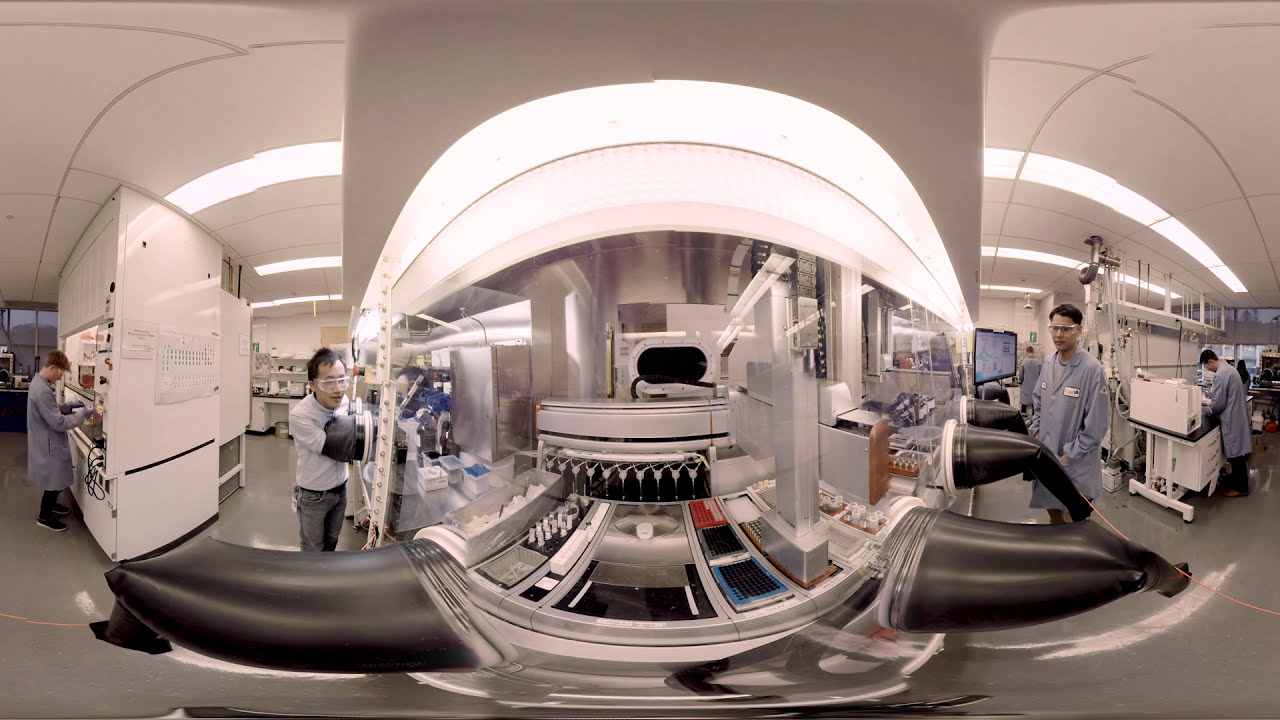The photo depicts a well-lit medical or laboratory setting featuring a large, complex medical device, possibly an MRI or CAT scan machine, prominently in the center. The machine has a clear glass window through which intricate internal components and trinkets are visible, illuminated by the light pouring from it. The image, likely captured with a wide-angle or 360-degree lens given its slight conical distortion, shows five professionals engaged in various tasks. On the left side, a man in a blue lab coat stands at a white workstation, while another person in casual clothing, donned with safety goggles, interacts with a blood pressure machine. On the right, two men in blue lab coats are seen; one peers at the machine while the other works at a desk. The facility appears sterile and scientifically equipped, emphasizing a high-tech, clinical atmosphere.